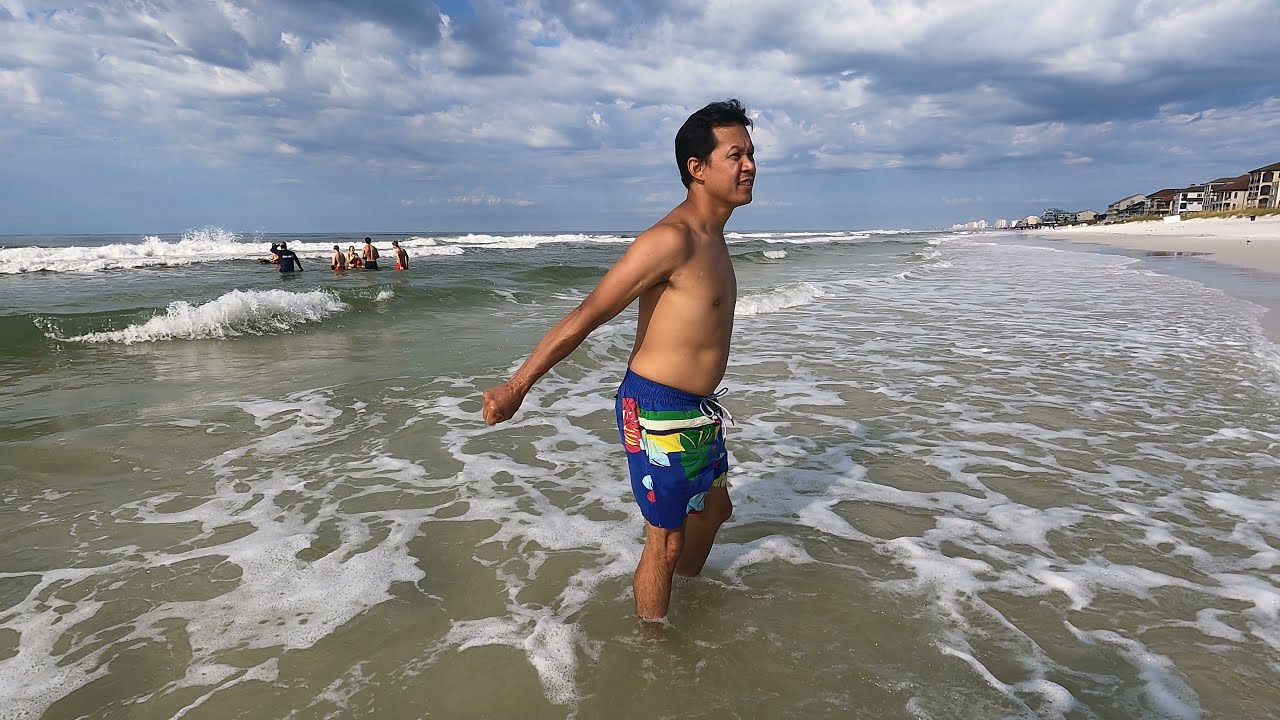In this outdoor beach scene, a shirtless man with short black hair stands ankle-deep in the ocean, wearing blue swim trunks adorned with green and red patterns. His body faces to the right, and he looks toward a sandy shore lined with houses and residential apartments in the background. The sky above is mostly gray, covered about 85% with a mix of dark and light clouds, indicating a partly cloudy day. Behind the man, about waist-deep in the water, is a group of indistinct people, possibly six, who are also wading in the waves. The ocean displays its dynamic nature with bubbling, foaming waves crashing on the shore. The image captures the lively and breezy ambiance of a daytime beach outing.